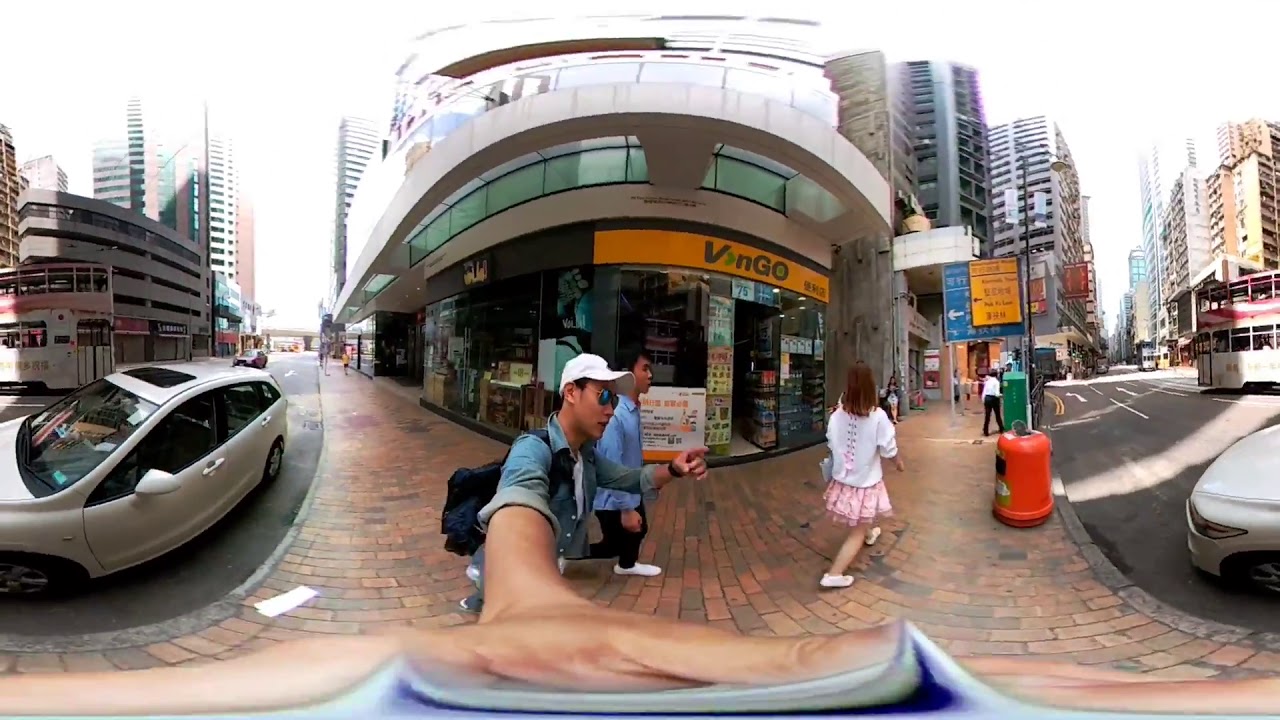In this vibrant panoramic image, a man stands in the center, captured in mid-walk on an orange-bricked pavement. He's sporting a white cap, blue sunglasses, a denim shirt with rolled-up sleeves, and a black backpack. His left arm, outstretched towards the edge of the image, holds the camera, creating a remarkable 360-degree view. Surrounding him is a bustling city street scene with a small, circular storefront directly behind him, bearing an orange banner with the text "Vingo" or "Vengo." 

To his left, another man in a blue shirt, black trousers, and white shoes walks alongside him, while ahead, a woman in a white jumper and pink skirt strides forward. Flanking the scene on both sides are parts of a white sedan; the left side showcasing its rear, and the right side its front. In the far background, tall buildings rise on either side of the street, encapsulating the urban atmosphere. Further detail includes a white double-decker tram visible on both sides of the image, a myriad of street signs in blue, orange, black, and yellow, and marked lanes, adding depth and motion to the cityscape.